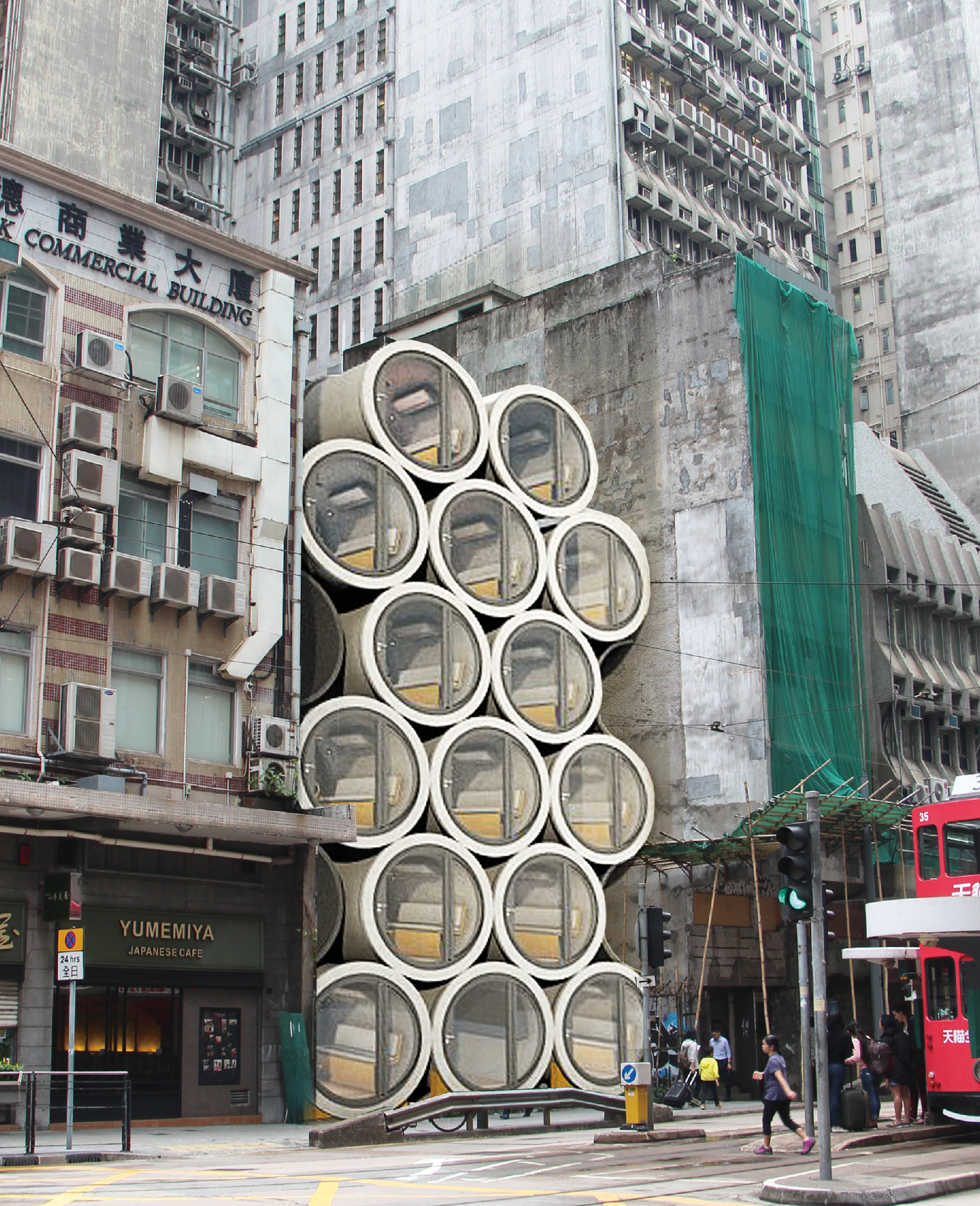The photograph depicts a bustling urban scene, likely in Japan, given the presence of signs with kanji characters and a "Yumima Japanese Cafe." The viewpoint is from street level, capturing a slightly diagonal alignment of buildings. Dominating the center is a notably curious structure consisting of capsule-like tubes with glass fronts, partially revealing interiors with yellow and white furniture. Adjacent to these capsules is a large commercial building adorned with numerous air conditioning units and a sign reading "Commercial Building." The buildings exhibit a gray, worn-down aesthetic. 

Pedestrians are scattered across the scene: a woman in a blue shirt and black pants walks from right to left, and a small group of three or four people can be seen further in the background. The lower left section features a distinctive red double-decker trolley, approaching the camera. To the right, a green curtain drapes from an adjacent gray building, adding a splash of color to the muted environment. Additionally, a green traffic light is visible below the curtain. The overall composition of the image captures the lively, yet somewhat aged, urban atmosphere.